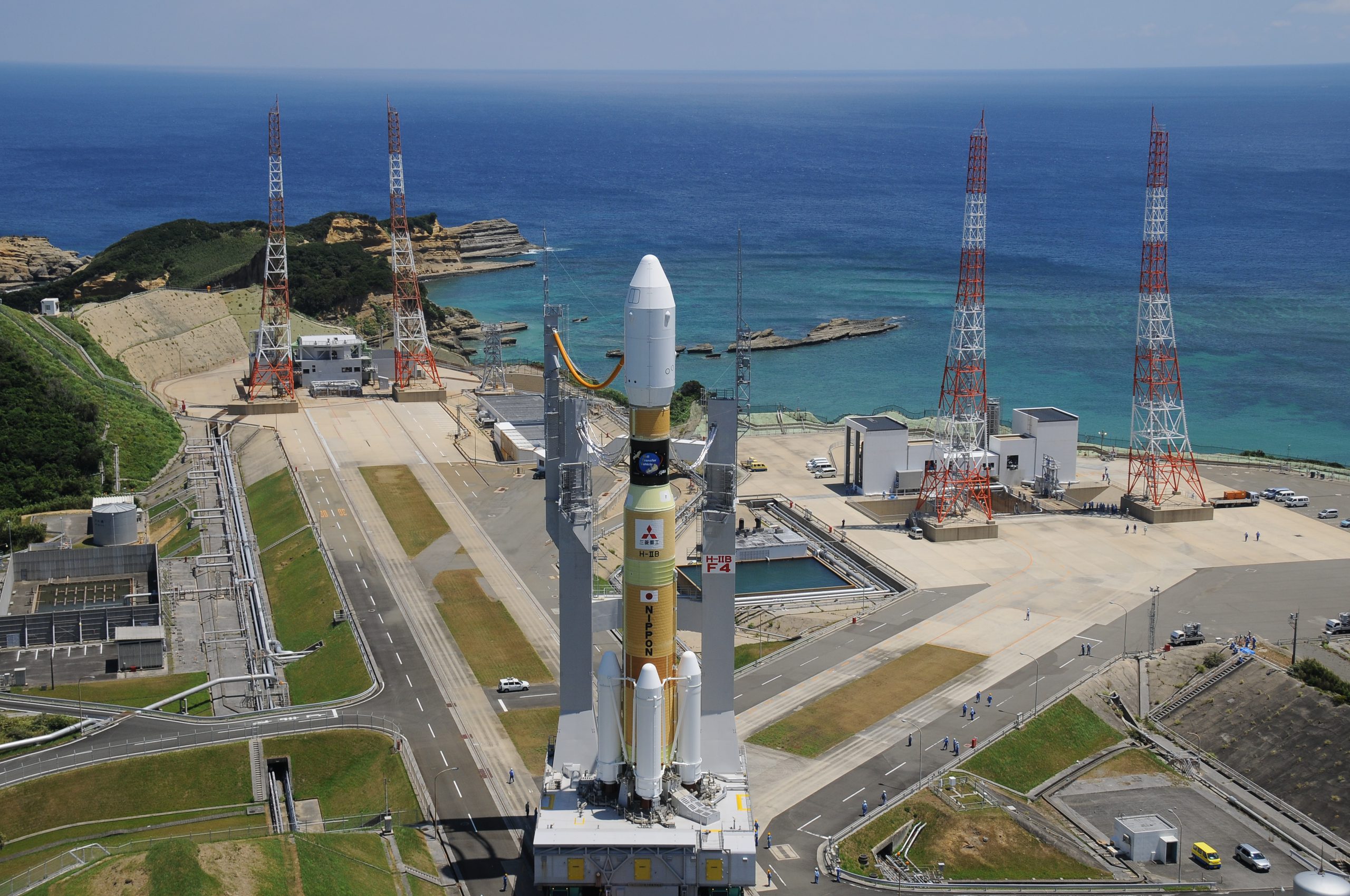This aerial photograph captures a detailed outdoor scene at a Japanese rocket launch site, likely depicting the Nippon space mission. Dominating the center of the image is a towering rocket standing on a gray concrete platform, ready for takeoff. The rocket features a distinct white nose cone with black and yellow bands, a red circle representing the Japanese flag, and the word "Nippon" emblazoned in black. The body of the rocket transitions into an orangish-yellow, connected to three large white fuel vessels at its base. The rocket is stabilized by two large gray towers flanking its sides.

Surrounding the launch platform is an intricate setup, including various infrastructure elements. To the left, an industrial building without visible windows stands amidst a patch of greenery. On the right, a sparsely populated parking lot with a few vehicles is observed. The area includes paved roads linking different sections of the site, with scattered people and several red and white transmitting towers or cranes visible in the background. 

The backdrop showcases an expansive, teal-blue ocean under a light blue sky, highlighting the site's coastal location, likely near Cape Canaveral-style launch infrastructure. The clear, vast waters and the serene sky frame the powerful rocket, enhancing the dramatic anticipation of the impending launch.